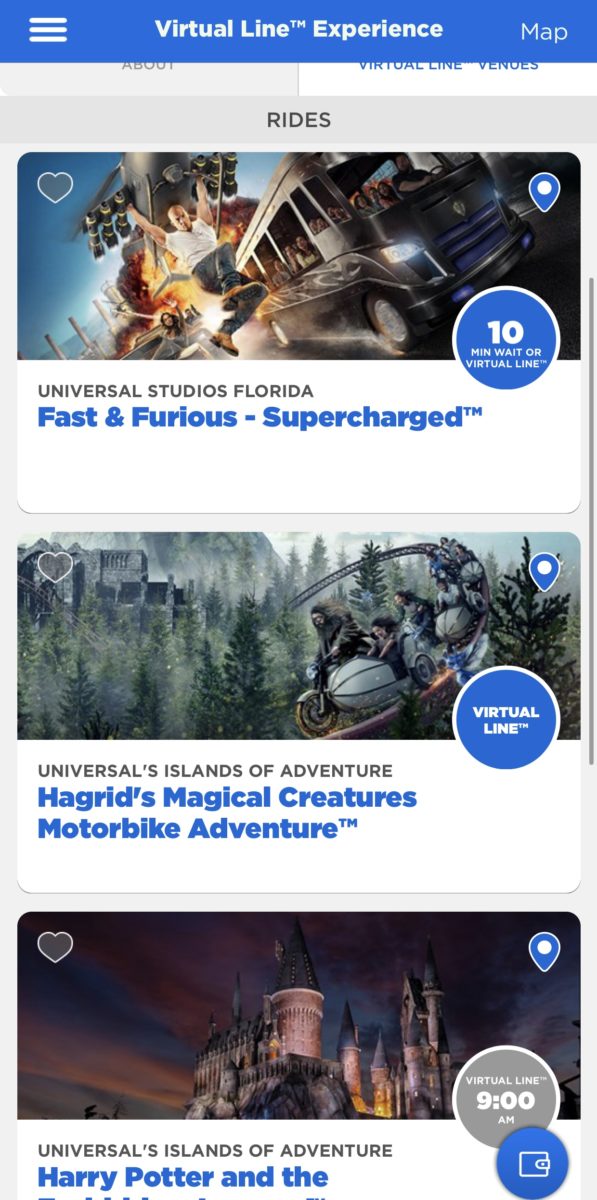The image showcases an elaborate visual map, predominantly surrounded by a light blue border. At the top, there's a deeper blue section featuring three small white lines accompanied by the text "Virtual Line Experience". The map prominently displays the word "Rides" against a light blue backdrop.

In the first section of the image, a ride from Universal Studios Florida titled "Fast & Furious: Supercharged" is highlighted. This section also features a small blue teardrop icon in the right corner and a circular icon with the number 10 in the center.

Further down, another ride is depicted with a similar blue teardrop icon alongside a white circle icon. This section includes a blue circle with words starting with "Virtual" and showcases "Universal's Islands of Adventure - Hagrid's Magical Creatures Motorbike Adventure."

The final section captures an image resembling the Disney castle. In this part of the image, a heart symbol is positioned in the upper left corner, while the familiar blue teardrop icon is present in the right corner. Additionally, there is a gray circle with the time "9:00," and a blue circle containing a square symbol. The text here starts with "Universal's Islands of Adventure - Harry Potter and the ..." but the remainder is cut off.